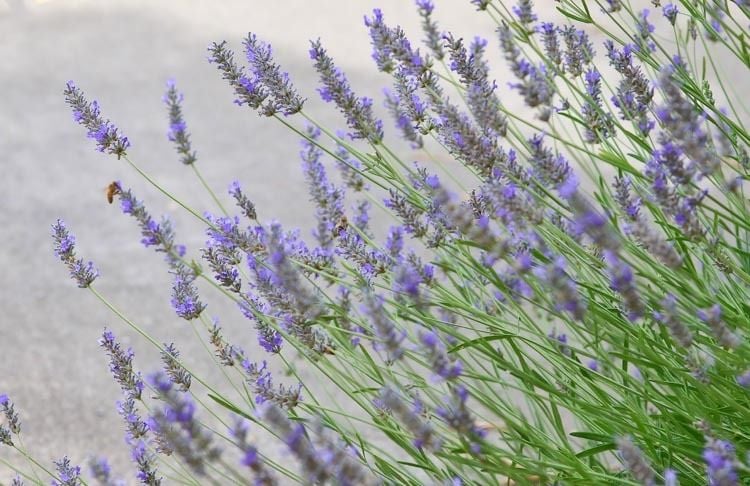This photograph captures a lush bush adorned with numerous purple clusters of flowers, resembling fox tails or potentially lavender. The bush features slender, elongated green stems that ascend diagonally towards the upper left corner of the image. Despite the slant of the picture, creating an illusion that the stems are growing from the bottom right, the focus remains predominantly on the vibrant flowers. The photograph zeroes in on these blooms, with the background being a blurred, cloudy sky, making the detailed and fully-bloomed flowers the center of attention. Additionally, a bee can be spotted perched on one of the flower clusters on the left side. The cropping of the image excludes the ground entirely, emphasizing the striking interplay of the green stems and the purple flowers set against the muted backdrop.